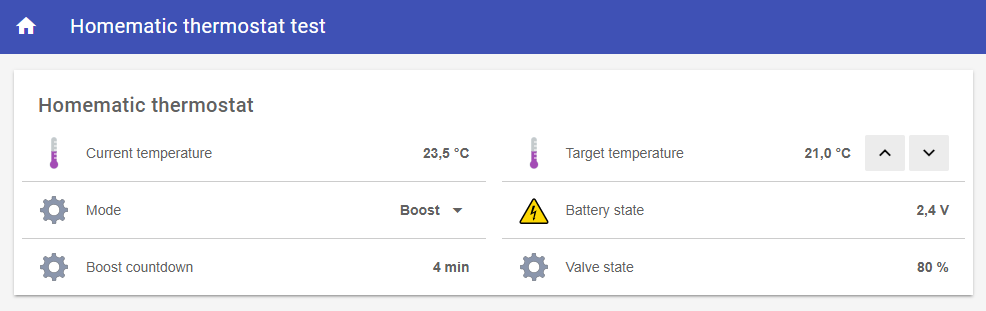A high-resolution image showcasing the detailed interface of a Homematic Thermostat Test. Positioned at the top of the display is a prominent blue section with a small white house icon located to the left. The rest of the interface is encased in a sleek, white box that provides comprehensive information about the thermostat's status. 

In the top section of the white box, the interface prominently displays "Homematic Thermostat." Below this title, the current temperature is shown using a classic mercury thermometer icon, indicating a precise measurement of 23.5°C. Adjacent to this, the heating target temperature is set and displayed as 21.0°C, flanked by intuitive up and down adjustment buttons for easy temperature control.

A subsequent section outlines the operational mode - currently set to "Boost" - adorned with a downward-pointing arrow symbolizing the active mode. Beneath this indicator, the battery status is conveyed by a yellow triangle featuring a lightning bolt, alongside the exact voltage of 2.4V. The interface also highlights a "Boost countdown" timer, which is currently set to 4 minutes remaining.

Lastly, the status of the valve is detailed with an icon resembling a cogwheel, indicating a valve state of 80%. This meticulous interface provides a thorough and easy-to-understand overview of the Homematic thermostat's performance and settings.